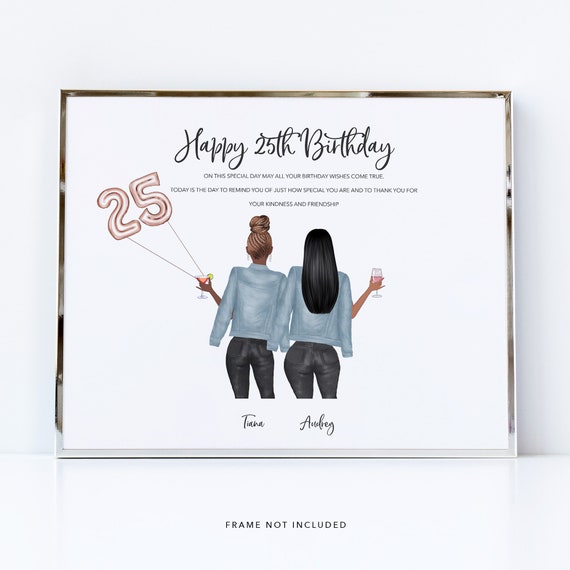This image depicts a piece of artwork designed as a special gift to commemorate a 25th birthday, presented against a white background with clear text indicating that the frame is not included. The artwork features two women named Tina and Aubrey, both dressed in matching blue denim jackets and black pants, celebrating with drinks in hand. The woman on the left, Tina, has her hair in a bun and holds a pair of balloons in the shape of the number 25, as well as a cocktail with a lime slice in a glass filled with a reddish-orange liquid. The woman on the right, Aubrey, has long, straight black hair and holds a wine glass containing a pink liquid. Above them, elegant black cursive text reads, "Happy 25th Birthday. On this special day, may all your birthday wishes come true. Today is the day to remind you of just how special you are and to thank you for your kindness and friendship." This celebratory and heartfelt message makes it a meaningful and thoughtful gift option for a friend’s milestone birthday.